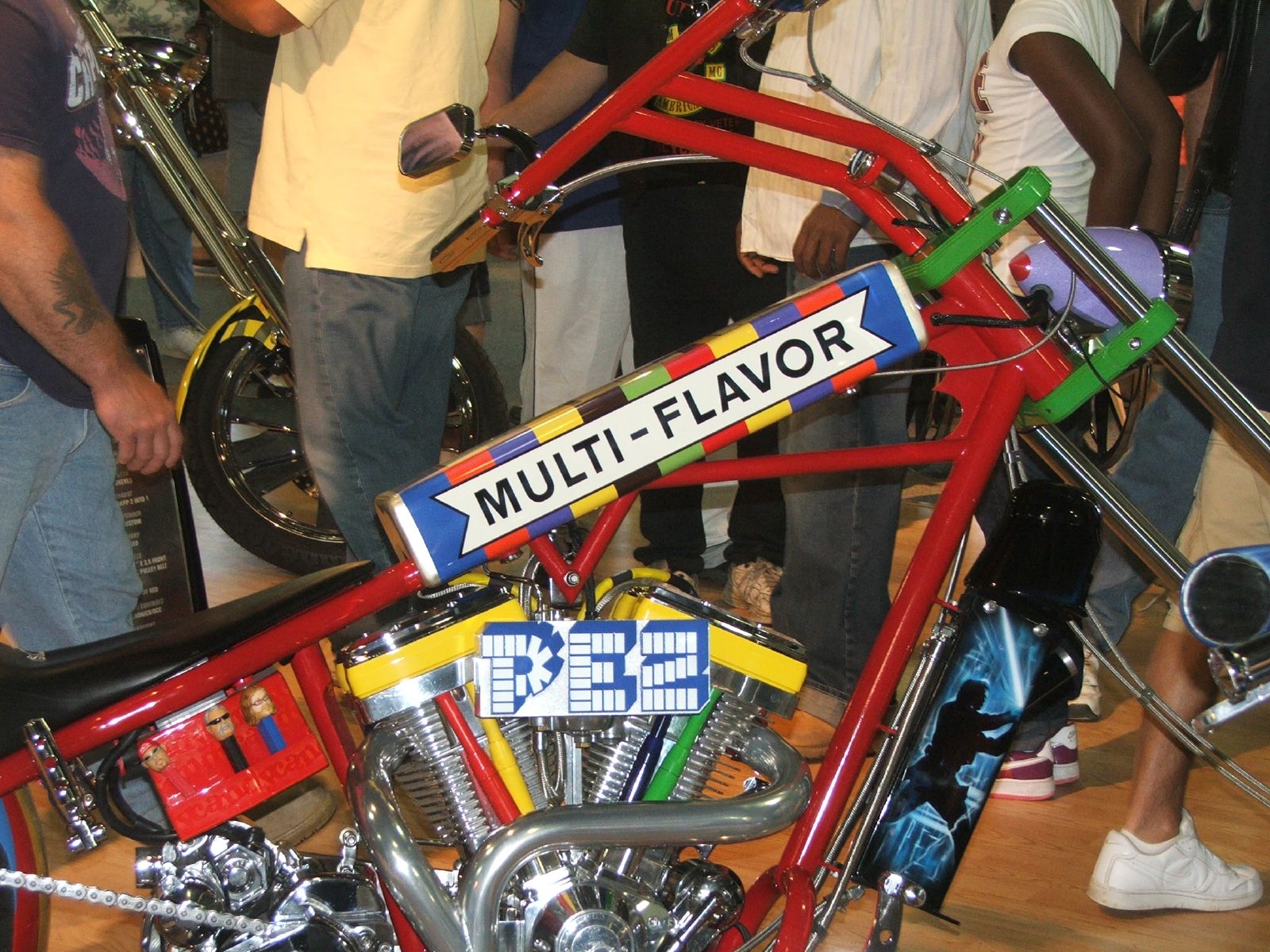This image depicts a custom-designed, glossy red motorcycle themed around the famous Pez candy brand, likely showcased at a motorcycle show. The central section of the bike prominently features the word "PEZ" in iconic blue and white lettering, mirroring the classic Pez candy font. Just in front of the black seat is a multi-flavor Pez pack, displaying an array of stripes in blue, red, yellow, black, and green colors. The handlebars are red, with additional green and silver accents around the front. The engine area is elaborately decorated with yellow, red, green, and silver hues, enhancing the festive, candy-like appearance. In the backdrop, several people are visible from shoulders down, suggesting a bustling environment with both spectators and other motorcycles faintly discernible.